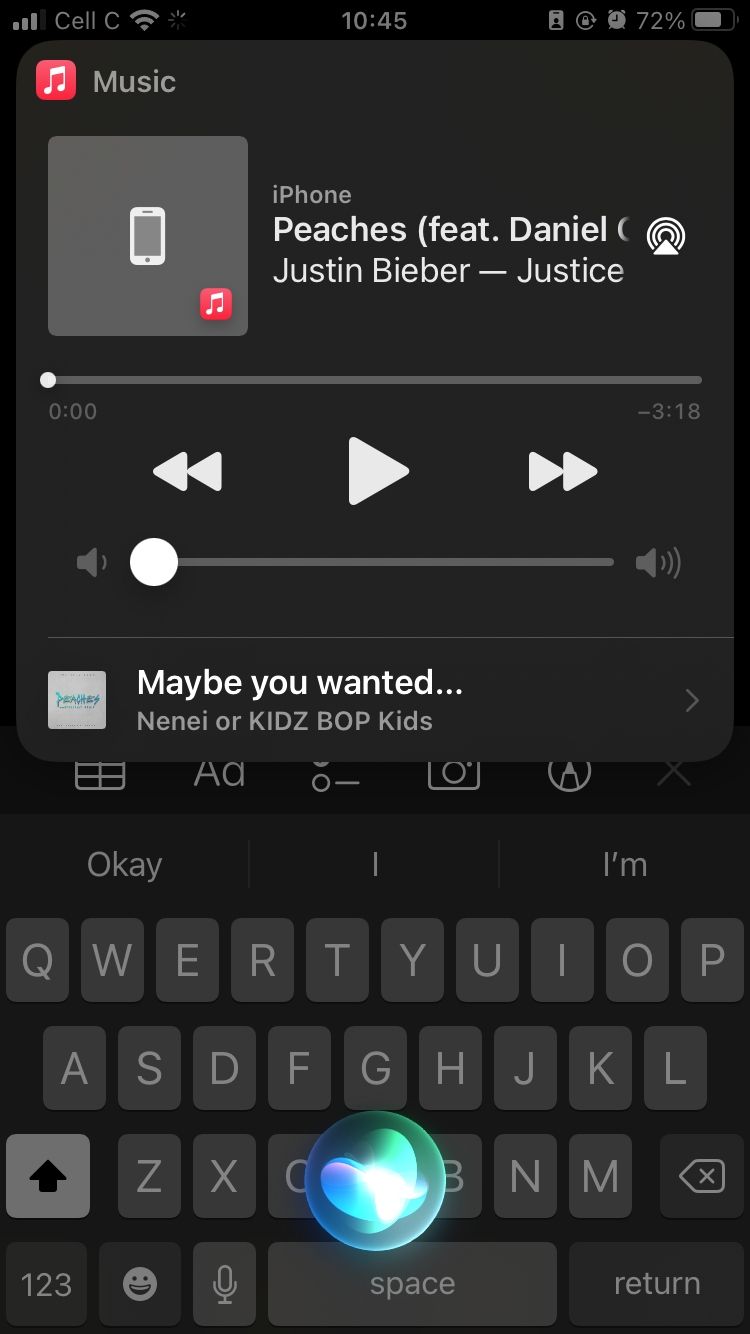The image is a screenshot from a smartphone. At the top part of the screen are several icons and indicators. Centered at the very top is the time, which reads 10:45. On the top right, there is an image icon next to the battery percentage showing 72%, followed by an alarm icon, a rotation lock icon, and a signal strength icon indicating the network provider is Celsius. Additionally, a Wi-Fi icon can be seen.

The main application open on the screen is a music app named "Pool Music" with a red and white logo. The screen displays the title "iPhone Pitches featuring Daniel Oh, Justin Bieber, Justice." A song is currently playing, although it is at the very beginning (0:00) out of a total duration of 3 minutes and 18 seconds. Below the song details, there are several control buttons including play, next, previous, and a mute button shaped like an envelope. 

At the bottom of the screen, suggestions like "Maybe You Wanted Nene" or "Kids Bop Kid" are displayed. The application features an advertisement from iTunes. The overall background of the image is black, with white text for clarity. A keyboard is present at the bottom of the screen, featuring a black background with grey key caps. On this keyboard, there is a Siri icon, along with the keys featuring a color spectrum including green, blue, and some other vibrant colors.